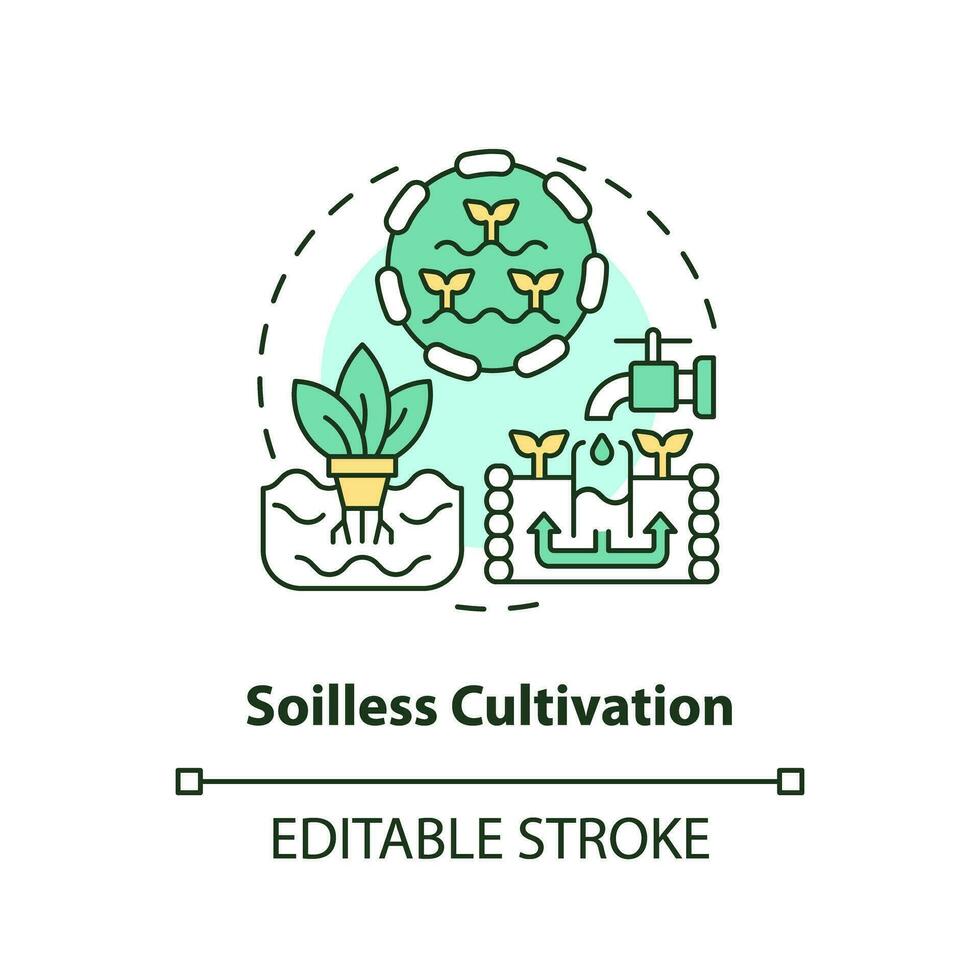This detailed vector graphic illustration, enclosed within a dashed black border, presents an informative and cyclical representation of plant growth. At the top, a spigot releases a single water droplet into the soil, symbolizing irrigation. Connected by two upward-pointing arrows, the water nourishes two seedlings growing in the ground. Moving along the cycle, a subsequent image depicts a plant pot containing a thriving plant with visible roots extending into the soil. Further along, a green circle outlined with white dashes contains three mature plants, symbolizing healthy growth. Below the illustration, bold black text reads "Soilless Cultivation," indicating a focus on alternative plant cultivation methods. Accompanying this is the phrase "Editable Stroke," aligned above a horizontal rule flanked by two small squares, suggesting the graphic's adaptability within image editing software. The combination of these elements forms a comprehensive visual narrative promoting the concept of soilless plant growing.